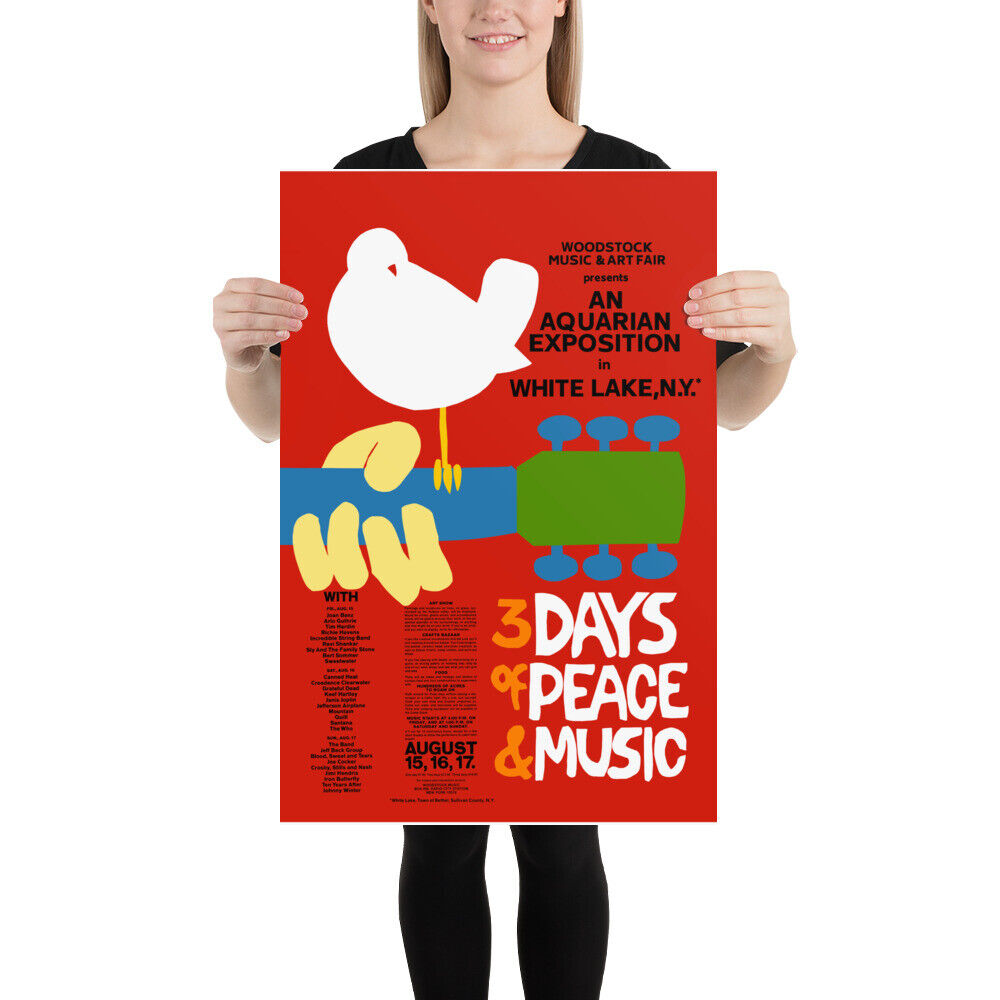A woman dressed in a black short-sleeved shirt is holding up a red poster for the Woodstock Music and Art Fair. The woman, whose face is cropped just above her nose, is smiling, and she has long blonde hair. The poster prominently features a white bird perched on the neck of a blue guitar, which also has a green head and blue tuning knobs, held by a yellow hand. The black text at the top reads "Woodstock Music and Art Fair presents an aquarium exposition in White Lake, NY." Below the guitar, it states "Three days of peace and music." On the left side of the poster, although largely illegible, are the names of the musical participants and the dates August 15, 16, and 17.